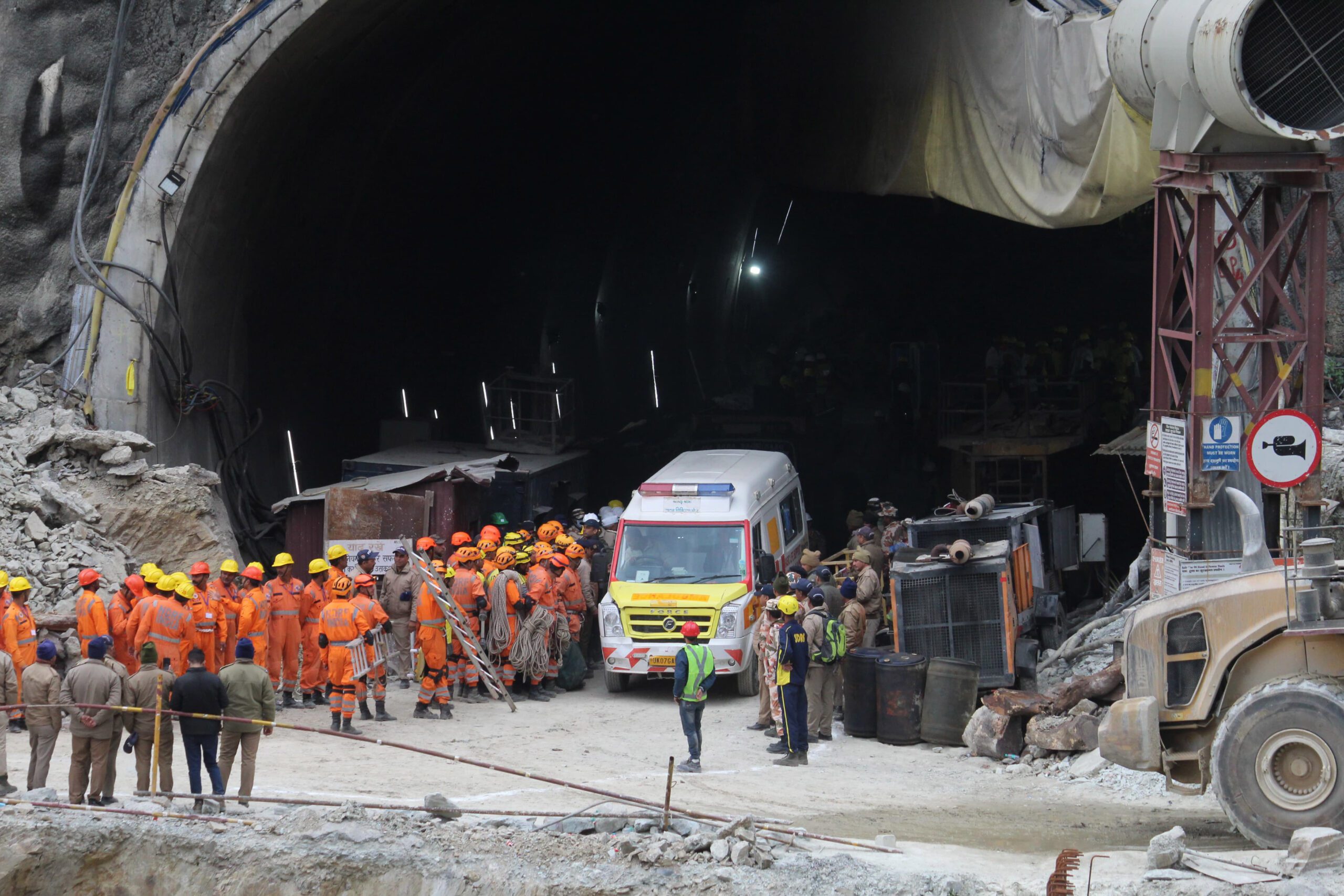This photograph captures an active construction site within a large, man-made tunnel structure. The arched, concrete walls of the long corridor give way to a dark, cavernous expanse, punctuated by small luminescent lights along the walls and numerous warning and caution signs. The bottom of the frame reveals a paved concrete surface scattered with a diverse group of workers. 

On the left, six men wearing gray jackets, gray khaki pants, and blue ball caps are visible. Adjacent to them, a cluster of workers in bright orange jumpsuits and a mix of yellow and orange hard hats are engaged in various tasks, such as carrying ladders and ropes. Dominating the center of the scene is an ambulance, marked by a yellow and white striped front, a white top, and red, white, and blue emergency lights.

To the right of the ambulance, more people in brown uniforms and a few in blue stand, one notably wearing a lime-green vest. The setting features an assortment of construction equipment, including three dark barrels and, on the far right, a large dusty machine with a substantial black wheel. Behind this machinery, red scaffolding supports a white circular vent, with black ducts stretching into the distance, contributing to the complex web of structures within the tunnel.